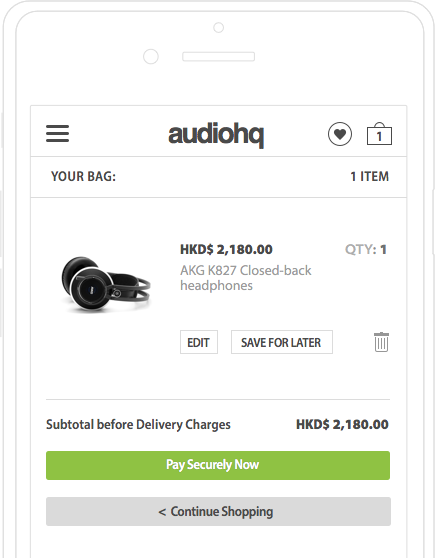**Detailed Caption:**

The image portrays a screenshot of a website named "Audio HQ," displayed on a simulated phone interface outlined in light gray. At the top center of the web page, "Audio HQ" is prominently featured in bold dark gray or black font. To the left of the website's title are three horizontal lines indicating menu options, while to the right, there are two icons: a circle containing a heart and a shopping bag with a numeral “1” inside it, all in matching dark gray or black hues. 

Below the site title, the active section is labeled "Your Bag," indicating one item present in the shopping cart. This section displays comprehensive details of the item: an image, the price, name, and quantity. The item listed is the "AKG K827 Closed-Back Headphones," priced at 2,180 Hong Kong dollars, with the quantity set to one.

Under the item description, there are functionalities to edit, save for later, or delete the item. A summary of the subtotal, excluding delivery charges, is also visible. To proceed with the purchase, a green box with white text offers the option to "Pay securely now," alongside a gray box with dark gray or black text suggesting, "Continue shopping."